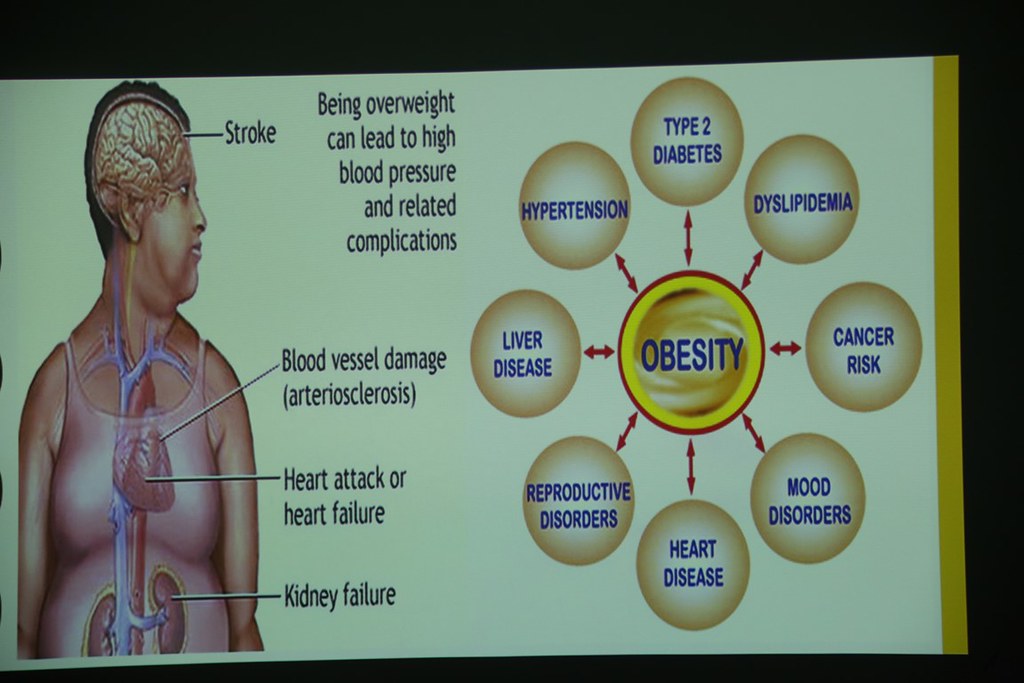This image appears to be a slide projected during a presentation, likely at a university or major educational institution, discussing the impacts of obesity. The left side features an anatomical illustration of a woman with visible internal organs and connections, showcasing how obesity affects different parts of the body. Black lines connect the brain, heart, and kidneys to labels indicating various medical issues: "stroke" for the brain, "blood vessel damage" and "heart attack or heart failure" for the heart, and "kidney failure" for the kidneys.

The right side of the slide contains a bubble map centered around the word "obesity" in blue letters. Arrows extend from this central bubble to other circles, each labeled with different conditions associated with obesity, highlighting a bidirectional relationship. These conditions include type 2 diabetes, cancer risk, mood disorders, heart disease, liver disease, reproductive disorders, dyslipidemia, and hypertension. The slide visually underscores the extensive health risks linked to obesity and emphasizes the interconnected nature of these conditions. The entire image is slightly canted, indicating it was likely captured from an angle rather than directly centered on the screen.